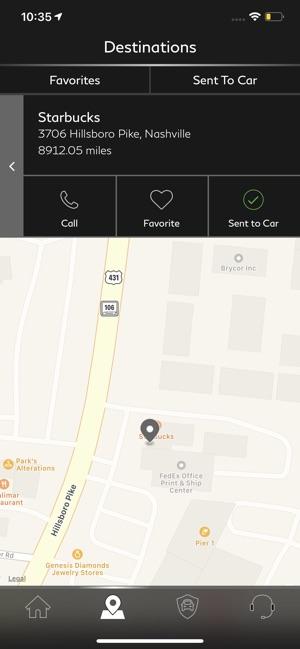This screenshot from a mobile website showcases a destination page, featuring a prominent black header labeled "Destinations." Below this header, there are two black tabs: "Favorites" on the left and "Sent to Car" on the right. Immediately beneath these tabs is a section dedicated to a specific Starbucks location. This section contains the name "Starbucks" in white font, followed by the address details. Adjacent to this information is a thin vertical gray panel with a left-pointing white arrow.

Underneath the Starbucks section are three black buttons: "Call" on the left, "Favorite" in the middle, and "Sent to Car" on the right, the latter marked with a green check mark. The main body of the screenshot displays a map with a pin indicating the location of the Starbucks.

At the bottom of the screenshot is a black navigation bar featuring four icons: a house icon on the far left, a location icon, a shield icon with a car, and on the far right, a headset icon.